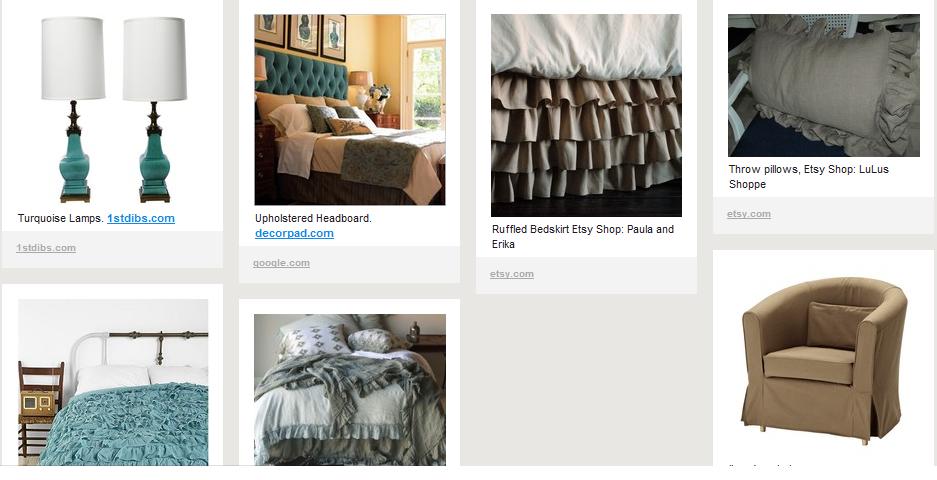This image is a detailed snapshot of a website showcasing various bedroom furniture products, all adhering to a cohesive design theme. The page includes multiple images of decor items. 

The first image features a pair of intricately designed bedside table lamps. These lamps have a vintage aesthetic, with bases crafted from a material resembling wood and finished in a turquoise hue. The lampshades are white, offering a striking contrast. A caption beneath the image reads "Turquoise Lamps," accompanied by a hyperlink to firstdibs.com.

The second image presents a fully furnished bedroom where these lamps would seamlessly fit. The bed features a turquoise upholstered headboard and is impeccably made, adorned with beige bedding, a white sheet, and a coordinating blanket. Three decorative pillows enhance the bed's appearance. Above the headboard, three turquoise-hued pictures are symmetrically arranged. The room is bright, with large, sunlit windows and walls painted in a light yellow-beige tone. A caption below this image reads "Upholstered Headboard," with a link to decorpad.com.

The third image showcases a ruffled bed skirt in a beige color, adding a touch of elegance to the bedding ensemble. The caption identifies it as a "Ruffled Bed Skirt," available on the Etsy shop Paula and Erica.

Additionally, there are four other images displaying items that complement the bedroom's color scheme and decor style, further emphasizing the cohesive design theme of the bedding and furniture collection.